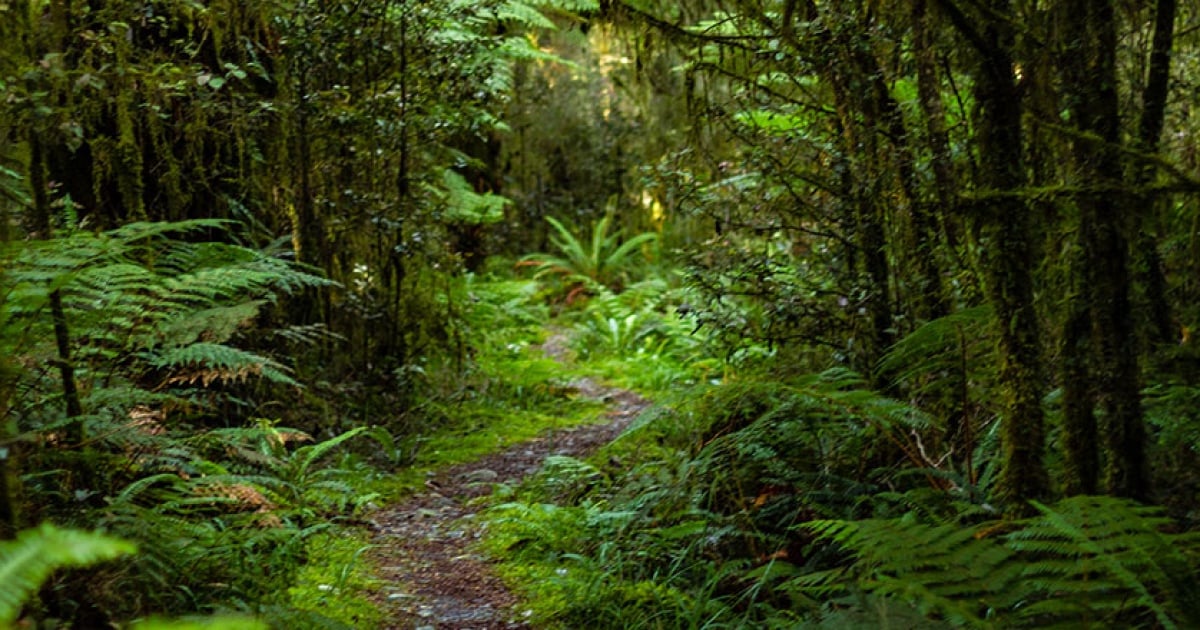This vibrant color photograph captures a lush forest scene, possibly a rainforest reminiscent of western Washington. Dominated by a rich green palette, the image showcases a narrow dirt path meandering in a zigzag pattern through the dense foliage. Both sides of the path are flanked by verdant ferns and large moss-covered trees. Though primarily shaded, a subtle glow of sunlight filters through the canopy, illuminating patches of the greenery and hinting at the daytime setting. There's no sign of flowers, animals, or people, focusing purely on the raw beauty of nature. A few leaves show a touch of orange, adding a slight contrast to the overwhelming green. In the background, a tiny hint of yellow light adds depth to the serene and untouched environment.